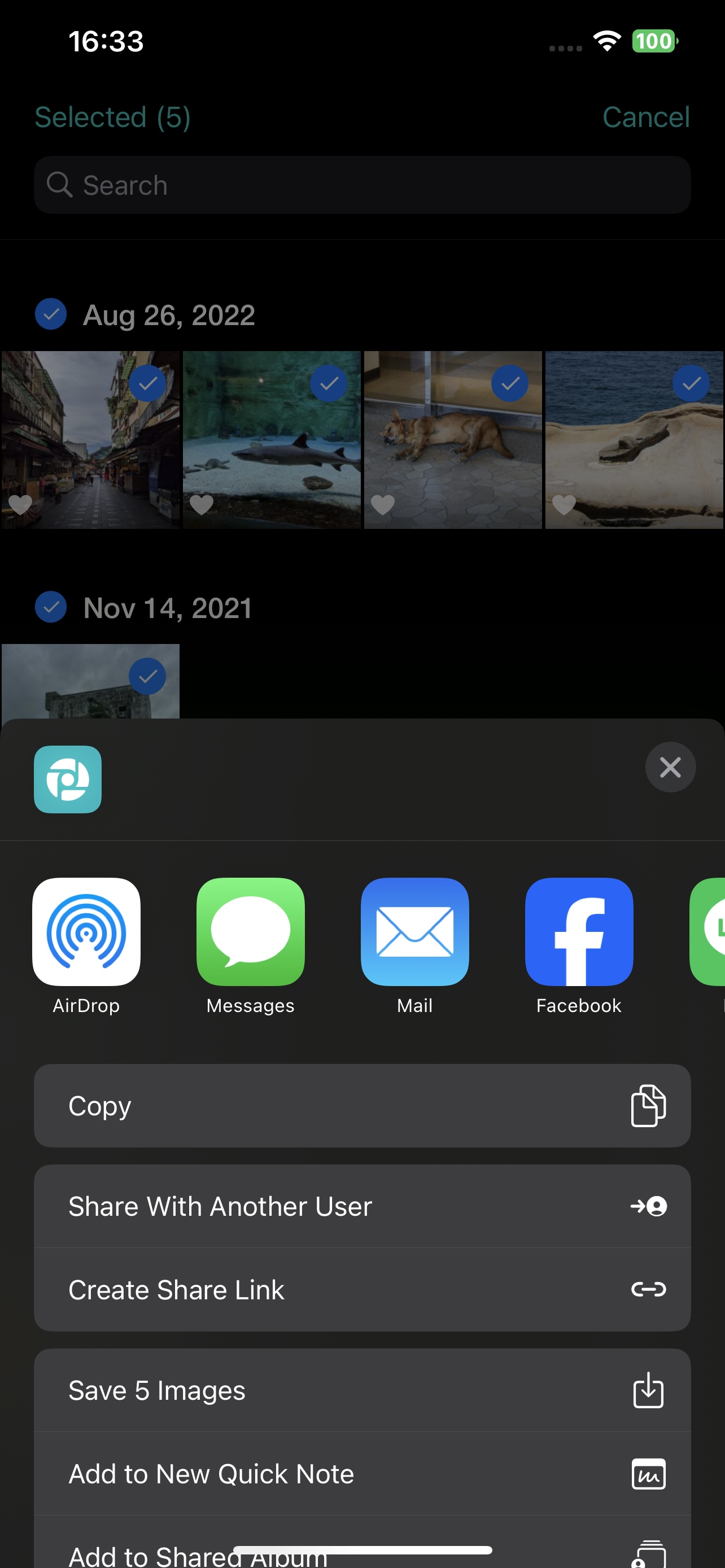The image is a detailed screenshot from the Photos app interface. At the top, there are thumbnail previews indicating selections of several photographs chosen by the user. Below the photo selection is a pop-up sharing bar displaying multiple sharing options. The first row of the pop-up bar includes icons and labels for several apps: from left to right, the options are AirDrop, Messages, Mail, and Facebook. The row below presents additional actions the user can take with the selected photos. The options listed in this second row are, in order: Copy, Share with Another User, Create Share Link, Save 5 Images, Add to New Quick Note, and Add to Shared Album. This comprehensive layout allows the user to quickly share or manage their selected images directly from the Photos app.